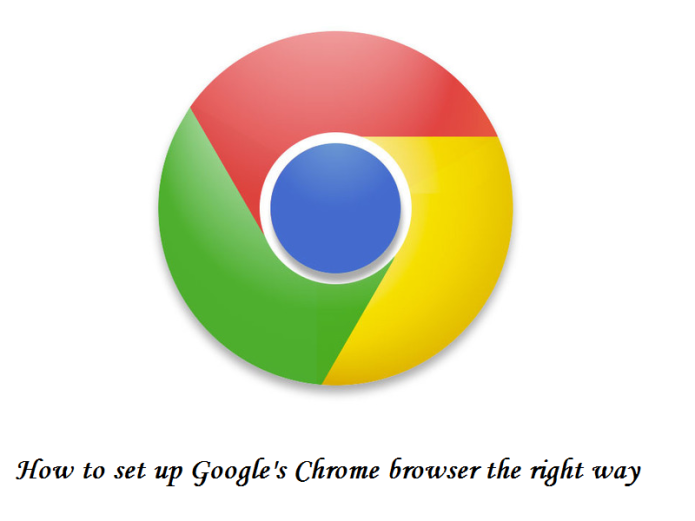The image prominently features the Google Chrome browser icon at the top. The icon itself is a complex, multi-layered circle. Starting from the outermost layer, it comprises three interlocking segments colored red, yellow, and green, creating a seamless loop of these three colors. Inside this tri-colored ring, there is a white circle which further encloses a smaller blue circle at the center, completing the recognizable Google Chrome logo.

Beneath this icon, the text "How to Set Up Google’s Chrome Browser the Right Way" is elegantly written in black italics, adding a touch of sophistication to the overall design. The text is straightforward, serving as a concise instructional tagline. The entire composition has a minimalist and attractive aesthetic, making it an ideal card for those looking to set up the Google Chrome browser effortlessly.